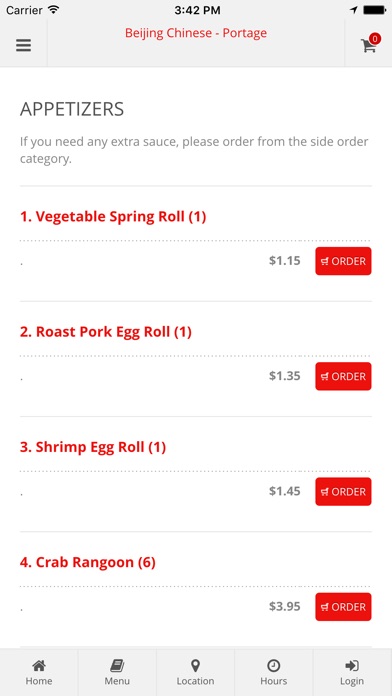The image features a user interface for a food ordering application on a mobile phone. 

At the top, there is a gray background with the word "Carrier" displayed in the left corner, and to the right, the time is shown as 3:42 PM. Below this header is the text "Beijing Chinese Portage" in a bold red font. To its immediate right is a black horizontal full battery icon, and next to it, a shopping cart icon with a small circle above indicating the number zero inside.

Directly beneath this, on the next line, is the section header "Appetizers." A small note below it states, "If you need any extra sauce, please order from the Side Order category."

The menu items are then listed vertically:

1. **Vegetable Spring Roll** (1 piece) - $1.15 
   - A red button labeled "Order" is on the right.
  
2. **Roast Pork Egg Roll** (1 piece) - $1.35 
   - Followed by another "Order" button in a red box on the right.
  
3. **Shrimp Egg Roll** (1 piece) - $1.45 
   - With an "Order" button placed to the right in red.

4. **Crab Rangoon** (6 pieces) - $3.95 
   - Accompanied by a similar red "Order" button on the right.

At the bottom of the screen, the standard navigation bar of the cell phone is visible, with options arranged horizontally: Home, Menu, Location, Hours, and Login.